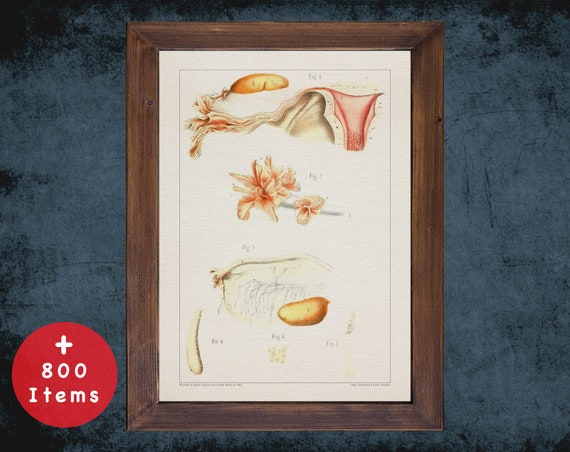The image depicts a framed piece of art with botanical illustrations that suggest anatomical forms. The artwork appears on a beige canvas-like material, framed in dark brown wood. The frame hangs on a backdrop of luscious blue velvet, with the corners shifting to black. Central to the piece, at the top left, is an illustration that resembles a uterus extending to a fallopian tube; this, however, transitions into more recognizable botanical elements—a pinkish-white flower in bloom, detailed meticulously in shades of rose and beige. Below this, various other indeterminate drawings add to the intricate array of the artwork. In the bottom-left corner, there is a prominent red circle, containing white text that reads "plus 800 items." The composition blends elements of anatomical illustration with botanical art, rendered with fine detail against a vibrant and textural background.